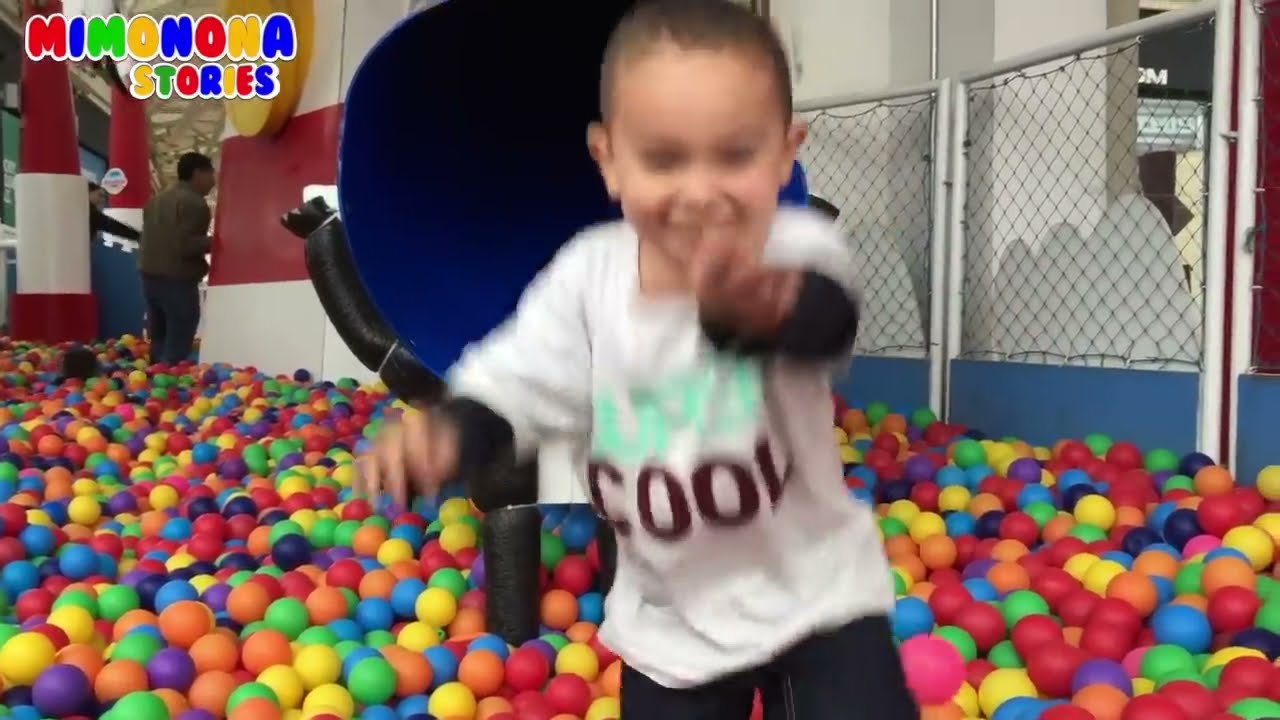In this lively image, a small boy, around four or five years old with very short brown hair, is caught in mid-movement, resulting in a slightly blurred effect. He is enthusiastically playing in a colorful ball pit, reminiscent of one in a Chuck E. Cheese or similar indoor playground. The boy is joyfully pointing directly at the camera with a big smile. He is dressed in a white t-shirt with light blue letters spelling out "cool" over a black long-sleeve shirt, paired with blue jeans. Surrounding him is a sea of small, multicolored balls, and behind him stands a blue slide, suggesting he may have just come down it. In the background, there is a red and white pole on the left side and a partition fence on the right, ensuring the safety of the play area. Also visible is an adult man, possibly a guardian, closer to the entrance of the ball pit, and a little girl playing beneath him. In the upper left corner of the image, multicolored bubble text reads "Memo Nona Stories," indicating this could be a screen grab from a playful video.